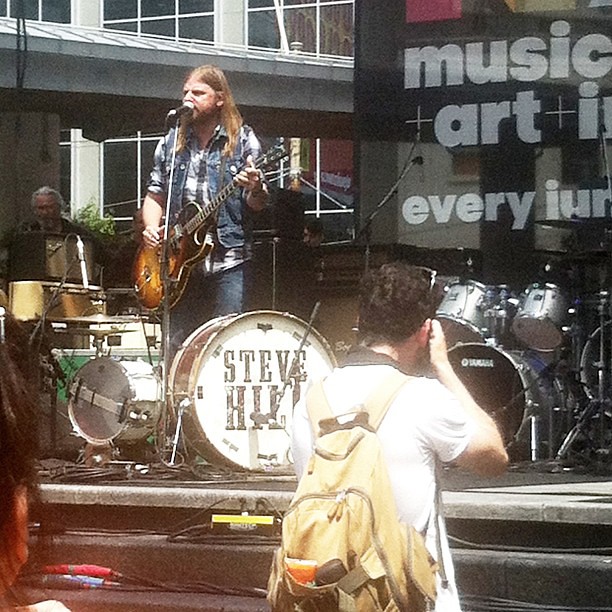The image captures a lively outdoor music festival held during the daytime, featuring a performance on a silver stage with a backdrop banner bearing the words "Music and Art." The focal point is a man with long brown hair, wearing a blue denim vest and blue jeans, passionately singing into a microphone while playing an electric guitar, likely a Gibson. The drum set beside him, marked with the name Steve Hill, stands prominent yet unmanned. The stage, festooned with various musical equipment, includes an older man in the background, possibly managing the soundboard. In front of the stage, a photographer with a yellowish backpack and a white short-sleeved shirt with sunglasses perched atop curly brown hair is seen capturing the moment. In the distance, a tall building, possibly a hotel, looms, adding to the festival's open-air ambiance.